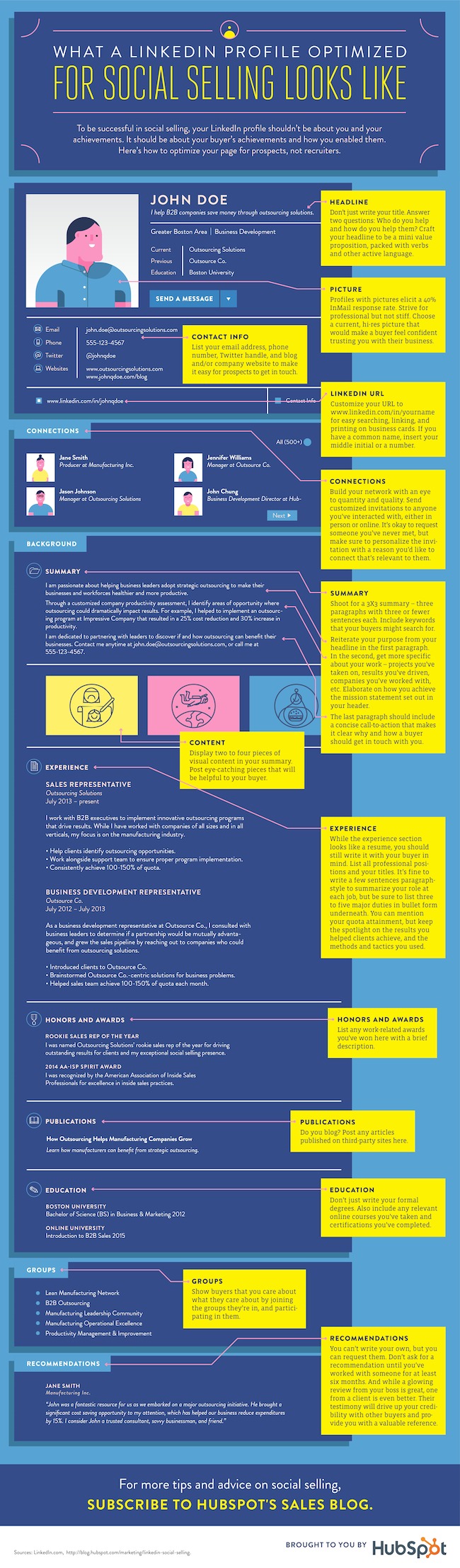This illustration is an intricate chart titled "What a LinkedIn Profile Optimized for Social Selling Looks Like." It features an illustration of a person labeled as John Doe, representing a generic LinkedIn user. Surrounding the central image are various sections of a LinkedIn profile, including 'Background,' 'Summary,' 'Experience,' 'Education,' 'Groups,' and 'Recommendations.' Yellow callout boxes provide detailed descriptions and optimization tips for each section, covering elements such as contact information, headline, and summary. While the text within the chart is small and hard to decipher, the main section headings are visible. At the bottom, there's branding information with logos and a call-to-action from HubSpot, encouraging viewers to "Subscribe to HubSpot's Sales Blog," indicating that this chart serves as both an educational tool and a marketing material to attract more users to HubSpot's resources.